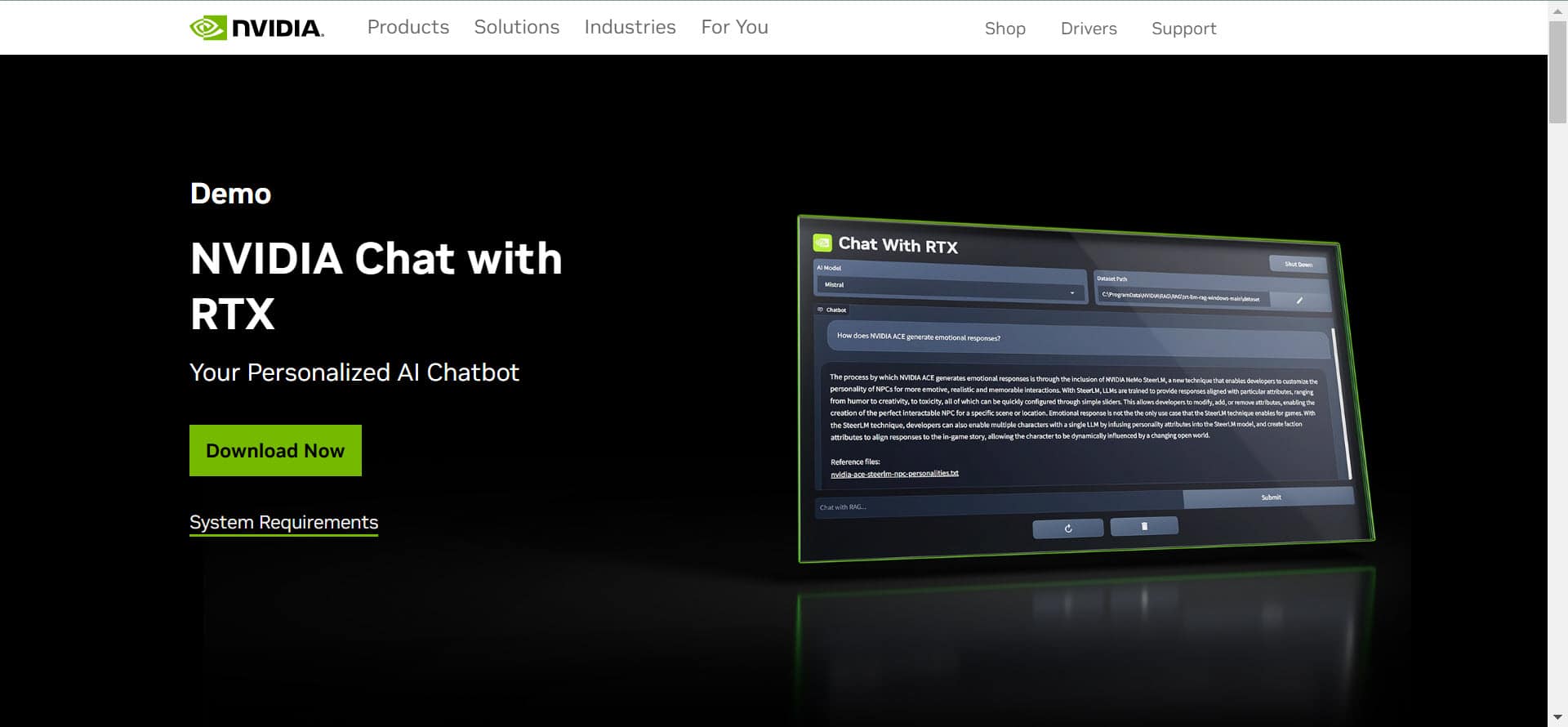This is a detailed screenshot from an NVIDIA website. In the upper left-hand corner, the green NVIDIA icon is prominently displayed beside the company name in all capital letters, "NVIDIA." Adjacent to the logo are the menu options in light gray: "Products," "Solutions," "Industry," and "For You." Further to the right are the additional menu options: "Shop," "Drivers," and "Support."

The main content area is dominated by a large black box. On the left side of this section, white text on a black background reads, "Demo NVIDIA Chat with RTX." Directly beneath this, in smaller white text, it says, "Your personal AI chat box," followed by a green button with black text that says, "Download Now." Below the button, white text with a green underline indicates "System Requirements."

To the right of this information is what appears to be a sample display of the product. The sample area is highlighted with a green outline against a black background and showcases the "Chat with RTX" interface. Several text boxes are available for typing prompts, and a large text box below these displays the response from the chat box. At the very bottom of the screenshot, smaller rectangular buttons are visible, possibly for additional actions or navigation.